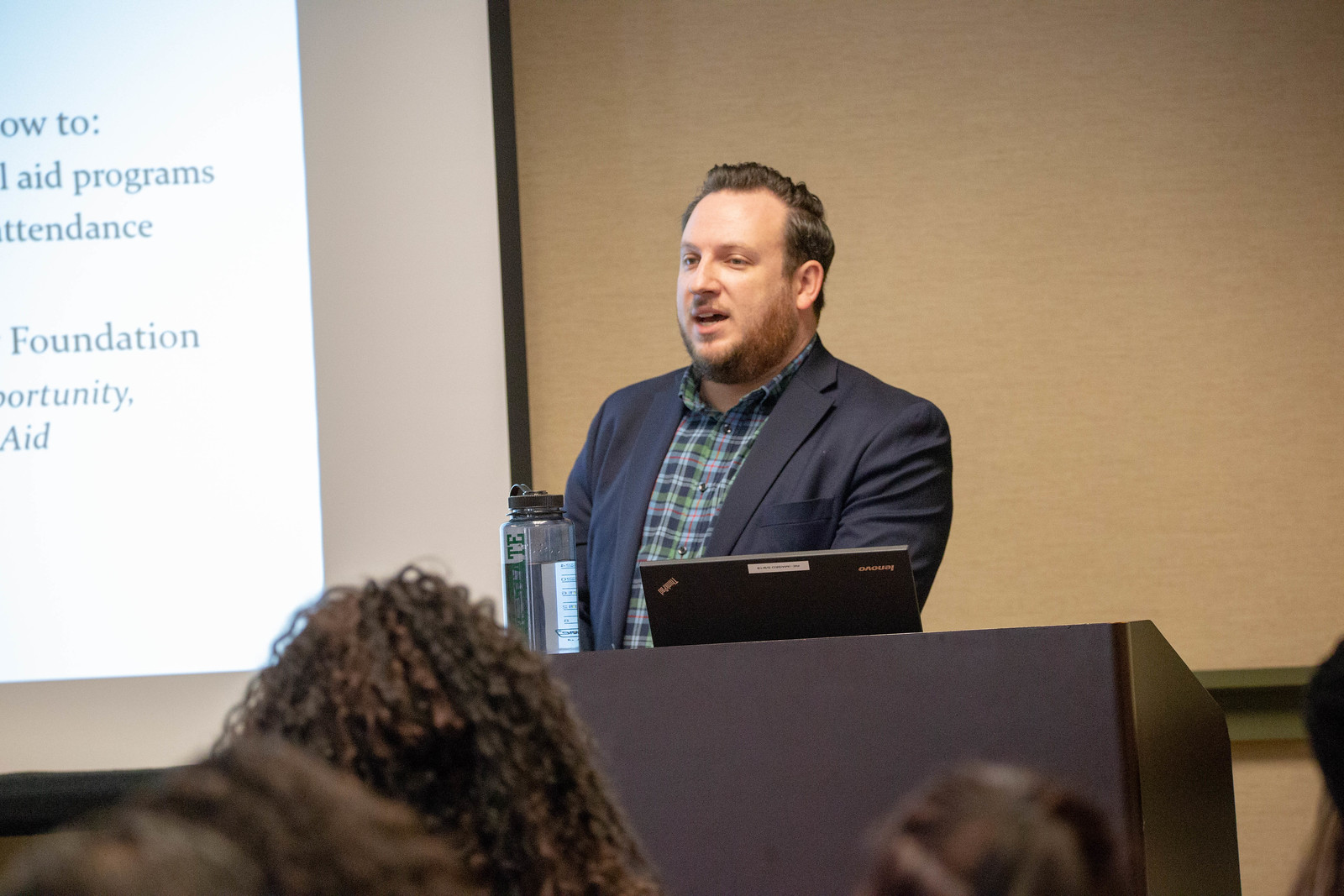In an indoor setting, likely a meeting or conference room with beige walls, a Caucasian man with a slight beard and brown hair stands behind a brown lectern. He wears a navy blue open sport coat and a plaid button-up shirt with white, blue, green, and red stripes. On the lectern sits an open Lenovo ThinkPad laptop and a clear plastic water bottle that is about three-fourths full, with a gray lid. The man is speaking to an audience, with his mouth open mid-speech and a projection screen behind him displaying partial text including words like "programs," "attendance," "foundation," and "aid." The audience, seated in front of him, consists mostly of individuals with dark hair. The image captures a professional and engaged atmosphere indicative of a lecture or presentation.